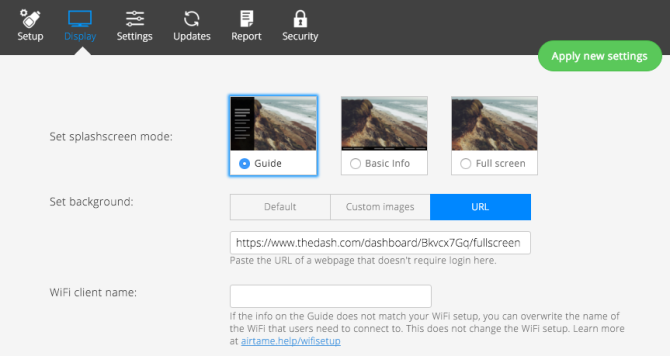The image is a screenshot from a computer displaying a settings interface. The top navigation bar is dark gray, with categories listed from left to right: Setup, Display, Settings, Updates, Report, and Security. The 'Display' category is highlighted in blue, indicating it's the current selection.

On the far right side, approximately halfway down between the gray top bar and the light gray background, there's a prominent green 'Apply New Settings' button with white text.

The main content area has a light gray background. On the left, in bold text, it reads 'Set Splash Screen Mode' with three available options: Guide, Basic Info, and Full Screen. The 'Guide' option is selected and outlined in blue.

Beneath this, there is a section labeled 'Set Background' with three choices: Default, Custom Images, and URL. The 'URL' option is highlighted, and underneath it, there's a text box containing a web address. This section is captioned with the instruction, "Paste the URL of a webpage that doesn't require login here."

Further down, there's an option labeled 'Wi-Fi Client Name' accompanied by an empty text box. Below the text box, additional instructions indicate, "If the info on the guide does not match your Wi-Fi setup, you can overwrite the name of the Wi-Fi that users need to connect to. This does not change the Wi-Fi setup." Furthermore, there's a blue hyperlink that says, "Learn more at www.airtame.help/Wi-Fi setup".